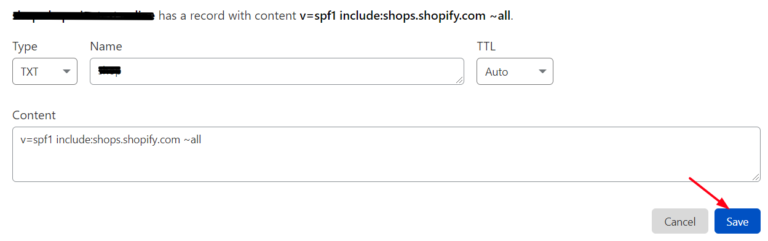The image features a section of an online form displayed against a white background. The top left corner has a few lines of text that have been obscured with a black strikethrough, rendering them unreadable. To the right of this, the visible text reads "has a record with content V=SPF1 include:shop.shopify.com -all".

Below this text, there's a labeled field named "Type" accompanied by a drop-down menu set to "TXT". To the immediate right is another field labeled "Name", but its content is also stricken through with a black line to prevent readability.

Further to the right, there is a segment reading "TTL" with a corresponding drop-down menu directly beneath it set to "Auto". Below this area, the form has a label "Content" followed by a text box containing the text "V=SPF1 include:shop.shopify.com -all". 

At the bottom of the form, there is a prominent blue "Save" button which is highlighted by a red arrow pointing towards it, indicating that this action should be taken.